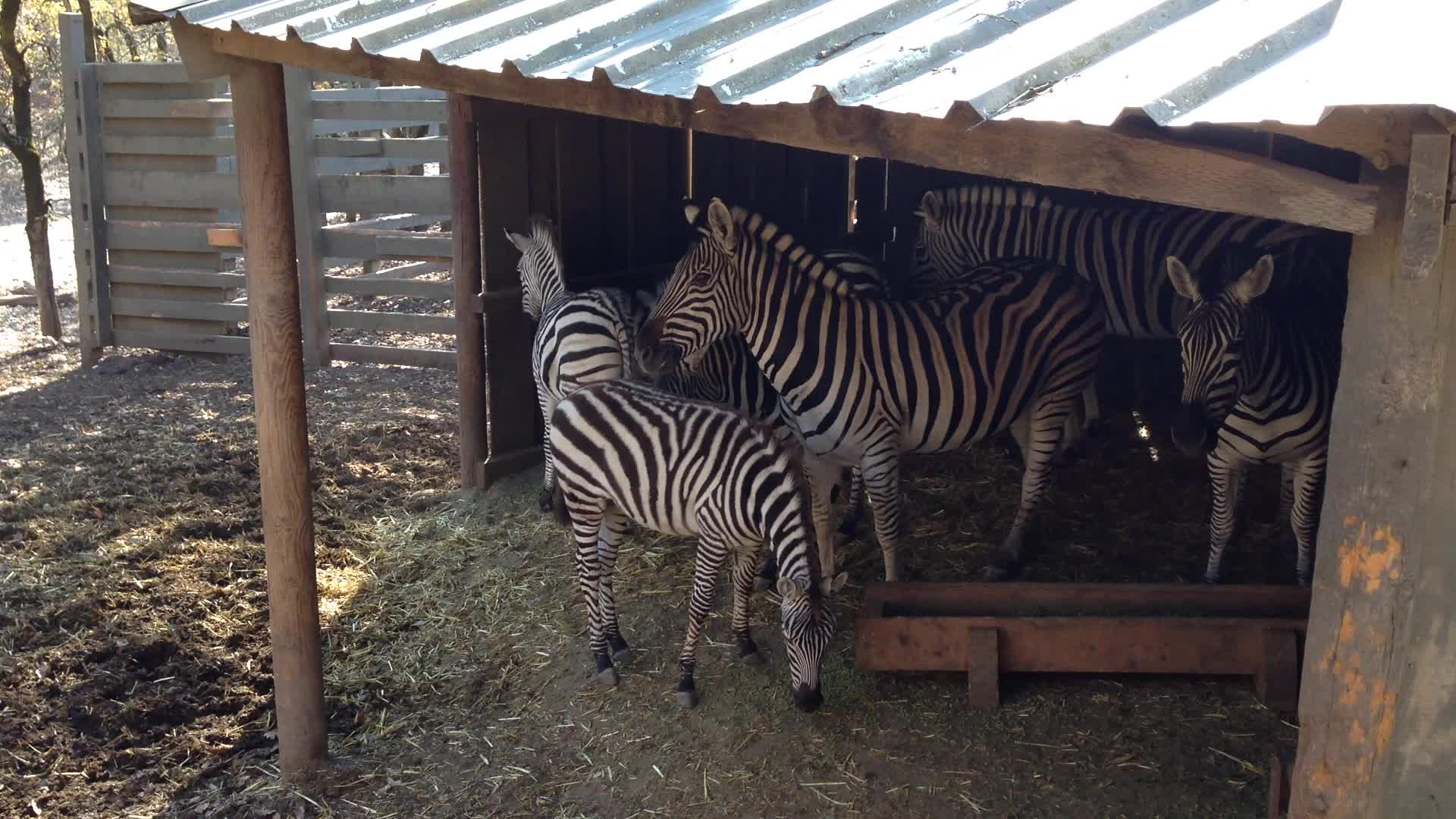This is an energetic color photograph capturing a small group of zebras – five in total – in what appears to be an open-air enclosure. The majority of the zebras are facing left and away from the viewer, with one distinctively facing towards the camera in the lower right-hand corner. These zebras exhibit traditional black and white striping and range in size, suggesting a mix of adults and younger zebras.

They are clustered closely together under a shelter with a galvanized metallic roof, supported by wooden posts on either side. The back part of the shed is enclosed, with small slivers of light peeking through the seams of the metal sheets. A large wooden gate with horizontal panels is visible in the upper right corner of the photo.

The ground beneath the zebras is a mix of grey dirt with patches of green grass, and scattered hay, indicating a well-used feeding area. A reddish object resembling a feeding trough with legs can be spotted at ground level. In the distance, trees are seen, and sunlight filters through, casting spots of light on the left side of the ground and the shed's roof, contributing to the dynamic atmosphere of the scene.